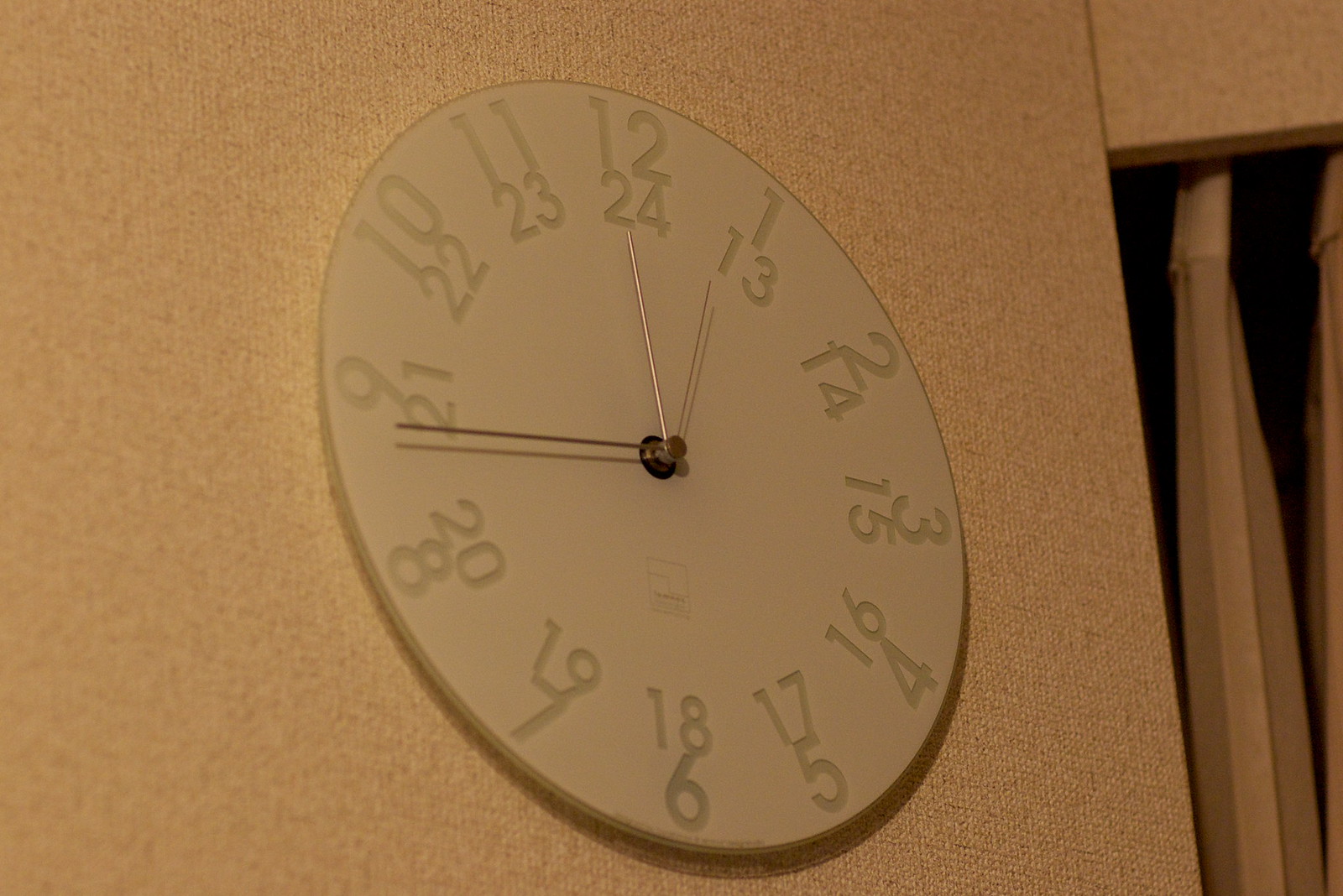The image captures a detailed view of a textured wall, resembling canvas material, in a light brown hue. On the right-hand side, there is a section of the wall that appears hollowed out, casting dark shadows within, with some indistinct brown elements hanging in the shaded area. Dominating the composition is a large pale green clock with hints of gray. The clock face displays conventional numbers from 1 to 12, accompanied by a complete set of military times from 13 to 24 beneath the standard numerals. The clock features an hour hand, a minute hand, and a second hand, all contributing to its detailed and functional design.